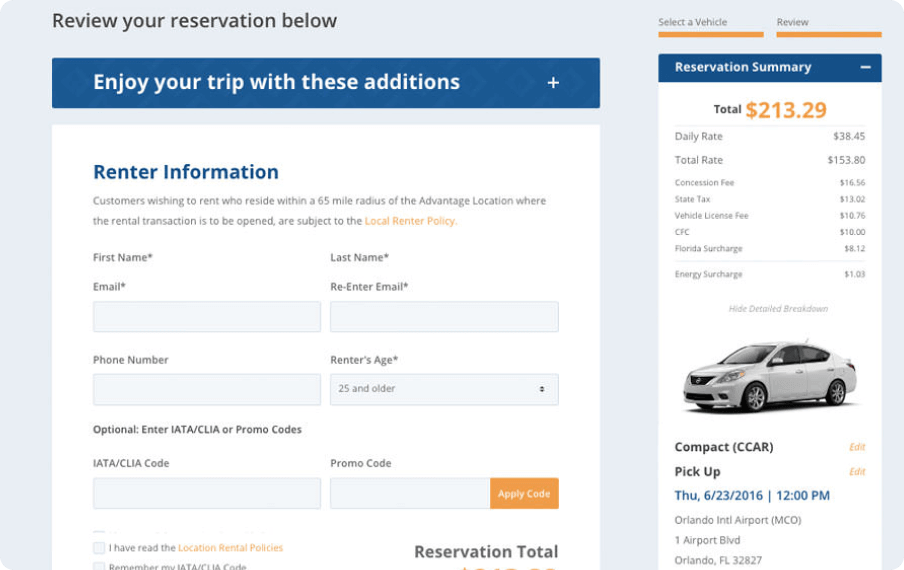**Detailed Caption:**

The screenshot showcases a rental booking interface, characterized by a streamlined and user-friendly design. At the top, a prominent blue strip runs horizontally with the text "Enjoy your trip with these additions" prominently displayed in white, standing out against the blue background. Below this, the primary section is set against a clean, white platform where users are prompted to enter their personal information.

In this section, "Renter Information" is written in bold blue text, with subsequent instructions and fields displayed in black font. Users must input their first name, last name, email address (and confirm it), phone number, and age. There is also an optional field for entering promo codes, should they have any.

Adjacent to these fields, a clickable yellow box with white text invites users to move to the next step. Nearby, there is another clickable box labeled "Select Vehicle," accompanied by a detailed reservation summary. This summary includes the total cost of $213, derived from a daily rate of $38, plus additional fees. The reservation specifies a compact car as the chosen vehicle, which is to be picked up on June 23. Additionally, a clickable link labeled "Local Renter Policy" provides further rental policy details.